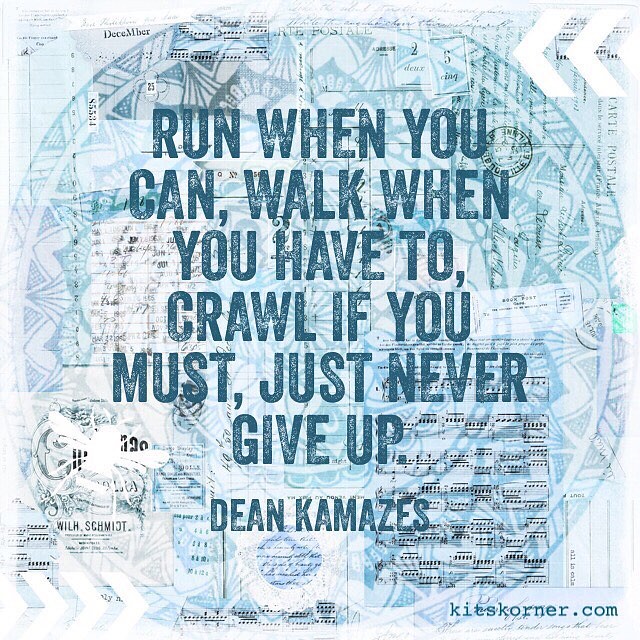This square motivational poster features a light gray background with a faint, light blue circular design at its center. The circle contains tribal-like markings, which are too indistinct to describe clearly, but evoke a sense of cultural motifs. Additionally, the background resembles a collage of documents, including elements that look like a round passport stamp with potential sun or flower icons in the center, white arrows pointing left in the upper right corner, and black sheet music with visible notes underneath, adding layers of texture.

Centered both horizontally and vertically within the circle, the distressed, all-capitalized text reads in darker blue: "RUN WHEN YOU CAN, WALK WHEN YOU HAVE TO, CRAWL IF YOU MUST, JUST NEVER GIVE UP." Below this quote, in similar but smaller distressed text, the attribution reads "Dean Karnazes," though there seems to have been some vocal ambiguity with the original spelling. At the very bottom right corner, in lowercase serif font, the website "kitskorner.com" is discreetly placed in blue.

This detailed layout of overlapping elements provides a rich visual and motivational experience aimed at inspiring persistence and determination.